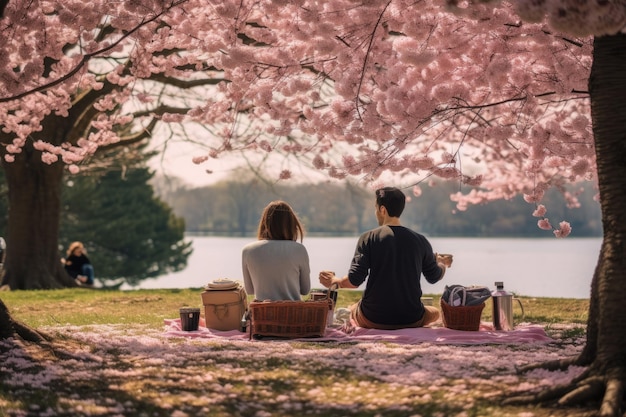In this serene springtime scene, a young couple enjoys a peaceful picnic under a canopy of blossoming pink trees. Captured from behind, the man, dressed in a black shirt and sporting short black hair, is seated on the right, while the woman with shoulder-length brown hair and a gray sweater sits on the left. They are comfortably settled on a pink blanket that has various picnic items around them, including two woven baskets, a large water bottle, and a pitcher with a liquid. The man appears to be gesturing as he talks, possibly holding a piece of their meal. Surrounding them, the ground is covered with fallen pink leaves, adding to the tranquil atmosphere. The couple gazes out over a calm body of blue water, which extends to a picturesque wooded area beyond. In the background, another woman sits under a tree to the left, with a pine tree standing behind her. The overall image is one of peace, warmth, and natural beauty, evoking a sense of calm on a lovely spring day.